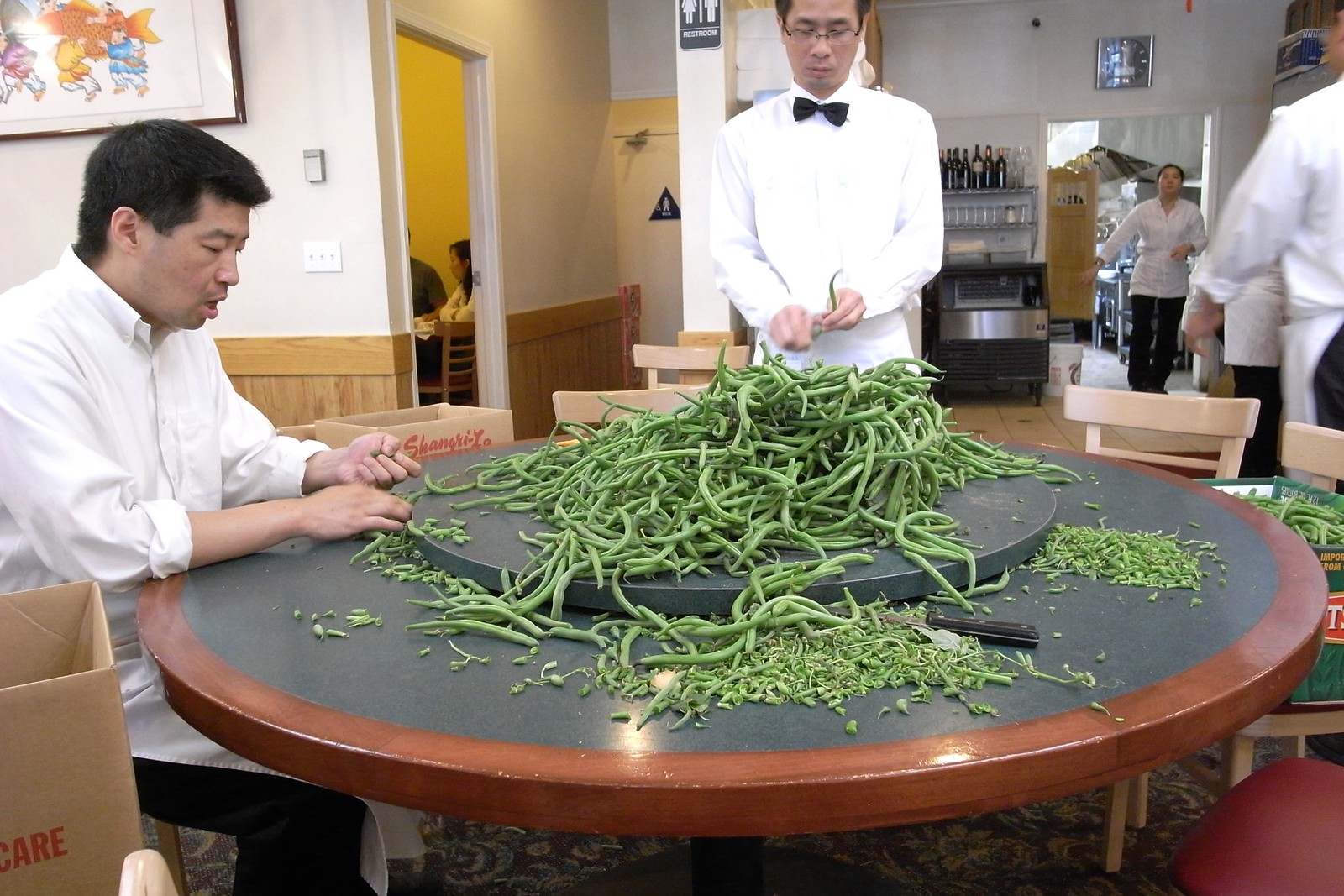In this bustling Asian restaurant kitchen, the scene is set with a large black-and-brown round table at its center, covered with a heap of green beans being meticulously sliced and cleaned by two men. Both men, dressed in white button-down shirts, one seated with an apron over his lap and the other standing donning a black bow tie, are deeply engrossed in their task. The kitchen’s backdrop reveals a stainless steel ice machine topped with wine bottles, contrasting against the half-white, half-wood paneled walls. To the left, customers are visible through an open doorway, enjoying their meals, while a woman in a white shirt walks towards the camera, emerging from what appears to be the back room. Additional kitchen staff can be seen moving about in the background, emphasizing the lively and organized chaos typical of a busy restaurant. A restroom sign is prominently displayed on a post, and a triangle symbol adorns another door nearby, adding further detail to this vivid depiction of a well-coordinated culinary space.